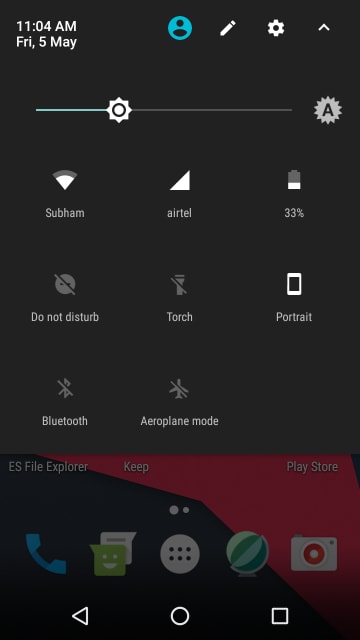This screenshot, taken from an Android phone, showcases the notification shade pulled down, revealing additional settings options. The phone is on the home screen, displaying a grayed-out background with partially visible app names. Prominent settings visible include adjusting brightness, toggling automatic brightness, and shortcuts for Wi-Fi, cellular data, battery status, Do Not Disturb mode, flashlight, screen rotation lock, Bluetooth, and airplane mode. While more settings are accessible by swiping right, they are not visible in this screenshot. The faintly discernible home screen background lists apps such as the Play Store, Keep, and a File Explorer. At the bottom of the screen, conventional app shortcuts are seen, including Phone/Contacts, Messages, and Camera. The top of the screen displays the date and time: Friday, May 5th, 11:04 AM.